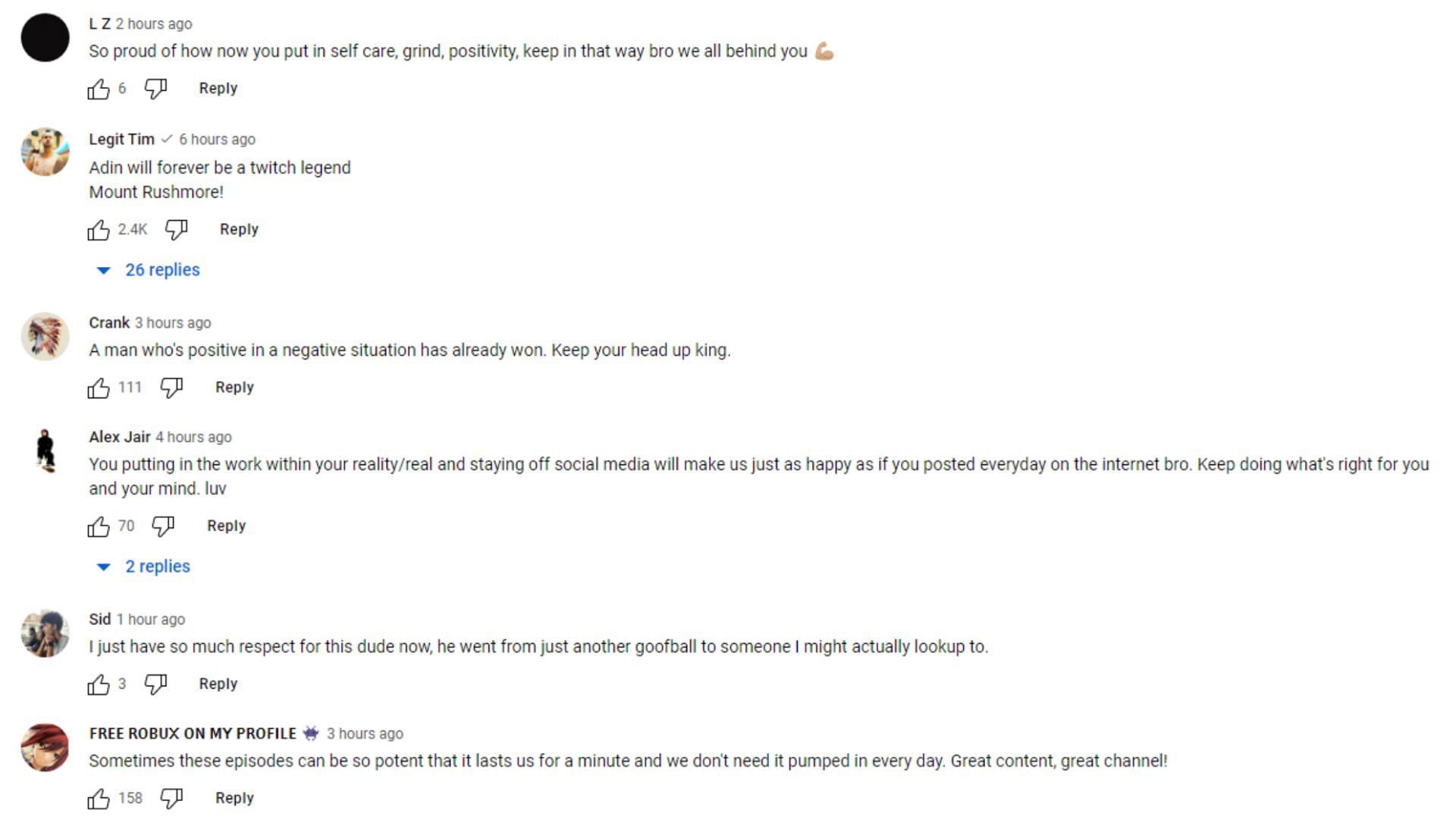The image displays a series of supportively engaged social media replies from six different users, offering encouragement and praise. The first user, LZ, writes, "So proud of how now you put in self-care, grind, positivity. Keep it that way, bro. We will all be behind you." Following this, Legit Tim comments, "Adam will forever be a Twitch legend, Mount Rushmore," which garners 26 replies. Crank contributes with, "A man who's positive in a negative situation has already won. Keep your head up, king." Next, Alex Jer remarks, "You putting in the work within your reality, real and staying off social media, will make us just as happy as if you posted every day on the internet, bro. Keep doing what's right for you and your mind. Love," receiving 2 replies. Sid adds, "I just have so much respect for this dude now. He went from just another goofball to someone I might actually look up to." Finally, Free Robux on my profile posts, "Sometimes these episodes can be so potent that it lasts us for a minute, and we don't need it pumped in every way. Great content, great channel."